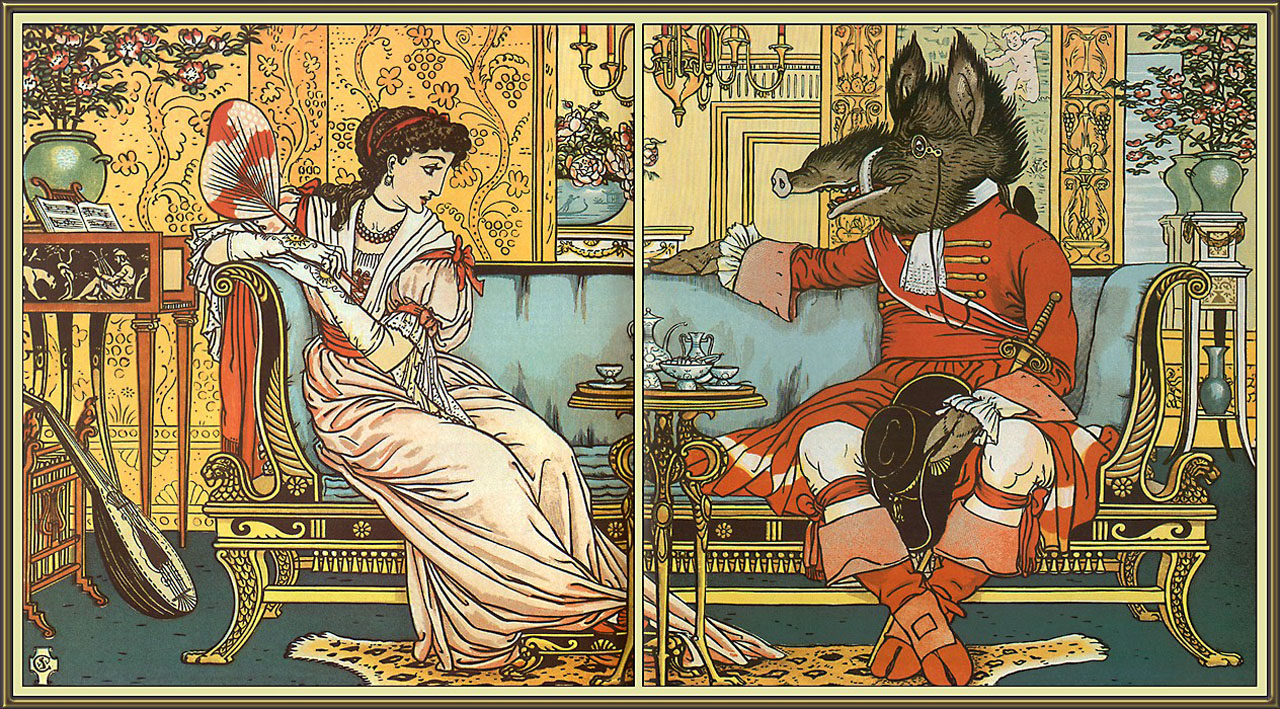The image is a detailed painting divided by a line into two sections. On the left side, there's an ornate room where a woman sits on a regal, blue chair. She wears an elegant, flowing peach gown that extends onto the right side of the image. Her hair is partially pulled back, cascading down her back. The room also contains a propped-up mandolin, a cabinet with a plant on top, and a possible crib in the corner. The woman gazes towards the right side of the image.

On the right side, there's an anthropomorphic figure with the head of a warthog, complete with a long snout, tusks, and an eyepiece. This creature, dressed in an orange princess costume and holding a hat, sits on a bench and makes eye contact with the woman. The hog-like figure's body is human-like but retains animalistic features such as hooves for feet. The scene is highlighted by a vibrant chandelier hanging from the ceiling, adding to the room's opulence. The characters’ attire and the room’s lavish decor create a whimsical and fantastical atmosphere.